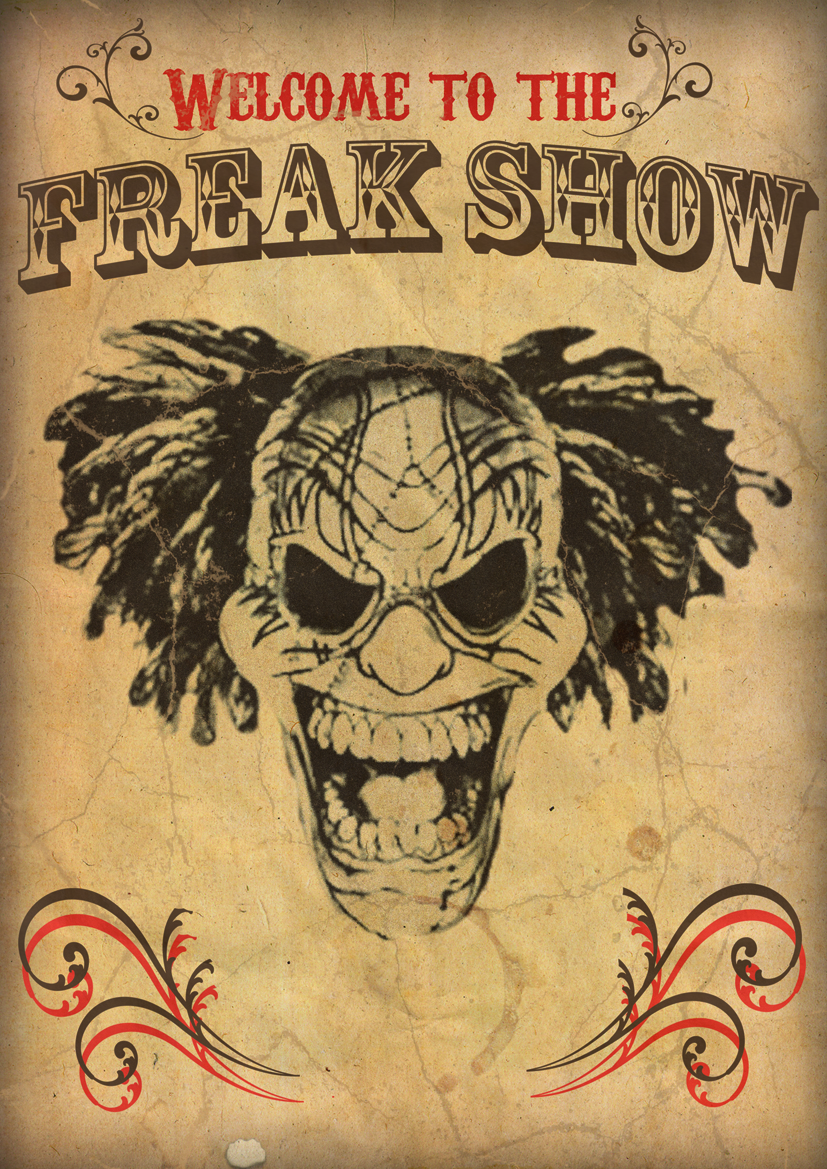The poster features an old-fashioned, highly detailed illustration with a vintage aesthetic. At the top, in bold red capital letters, it declares "Welcome to the," followed by "Freak Show" in prominent black and pale capital letters. The background is a light brown with a worn, crackled texture, enhanced by ornamental scroll designs in both the bottom left and right corners. Dominating the image is a menacing clown with a ghastly expression. The clown’s face is characterized by a wide, unnerving grin that reveals all its teeth. It has wild, fluffy hair that erupts from the sides of its bald head, reminiscent of a mad scientist's disheveled locks. The clown wears sunglasses that obscure its eyes, leaving dark, hollow sockets visible. The overall appearance of the clown exudes a combination of chaos and menace, brilliantly capturing the eerie essence of the "Freak Show" theme.